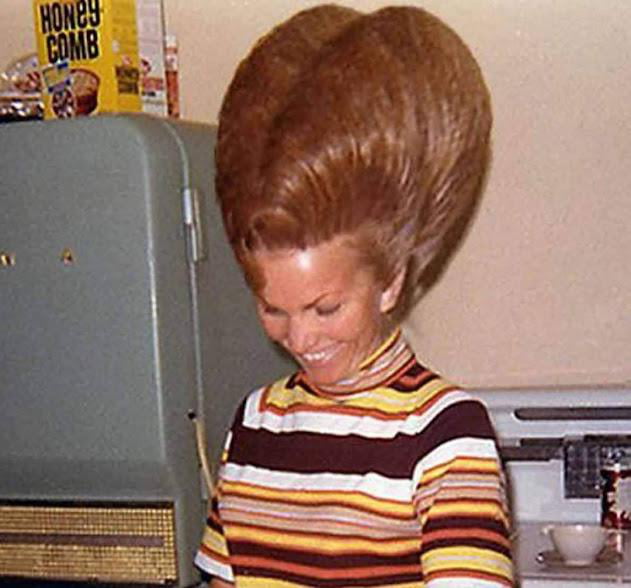The image appears to be a nostalgic photograph from the late 1950s or early 1960s. It features a woman with an elaborate and voluminous hairstyle, reminiscent of two thick fins positioned atop her head. She is bending slightly forward, gazing downward with a gentle smile on her face and her eyes partially closed. She is dressed in a boldly striped shirt featuring a mix of brown, white, yellow, and orange colors.

The woman is positioned next to an old-fashioned refrigerator, distinctively metallic gray with a prominent thick gold band in its midsection, indicative of the appliance design during that era. Atop the refrigerator, there are two boxes, one of which is identifiable as Honeycomb cereal. In the background, partially visible, is either a stove or a table with a coffee cup placed on it, adding a homely touch to this vintage scene.